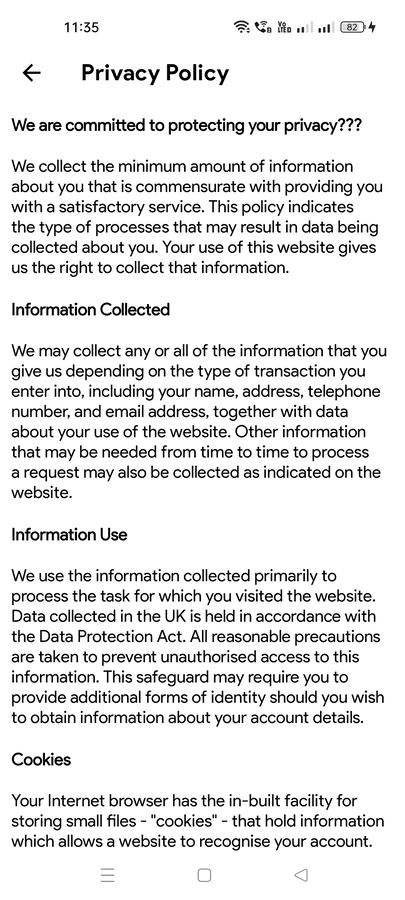This is a detailed screenshot from an Android phone, recognizable by its home menu which includes a home button, back arrow, and three lines at the top. The time displayed is 11:35, and the battery life is at 82%. The screenshot captures a privacy policy page.

At the top of the page, there's a heading that reads, "We are committed to protecting your privacy," in bold black text. Following the heading, the first paragraph explains, "We collect the minimum amount of information about you that is commensurate with providing you with a satisfactory service. This policy indicates the type of processes that may result in data being collected about you. Your use of this website gives us the right to collect the information below."

The subsequent section titled "Information Collected" states, "We may collect any or all of the information that you give us, depending on the type of transaction you enter into, including your name, address, telephone number, and email address, together with data about your use of the website. Other information that may be needed from time to time to process a request may also be collected as indicated on the website."

The next section, "Information Use," elaborates, "We use the information collected primarily to process the task for which you visited the website. Data collected in the UK is held in accordance with the Data Protection Act. All reasonable precautions are taken to prevent unauthorized access to the information. The state government may require you to provide additional forms of identity if you wish to obtain information about your account details."

At the bottom of the page, there is a mention of "cookies."